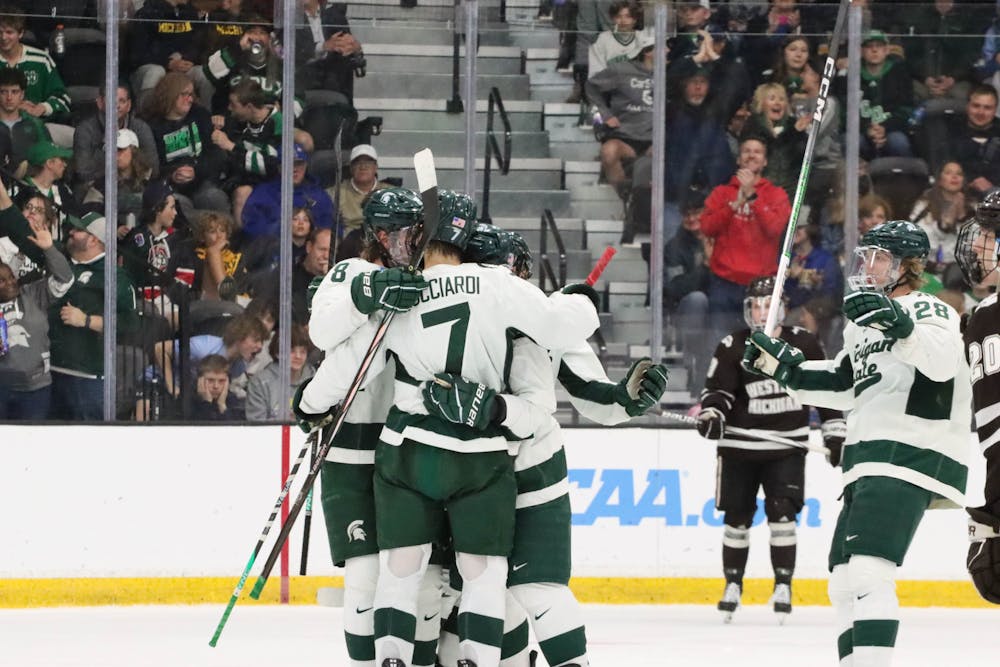This photograph, captured on the rink itself, showcases a thrilling moment from a college hockey game featuring the Michigan State Spartans and the Western Michigan Broncos. In the foreground, three to four male Michigan State hockey players, dressed in green and white, are seen embracing each other in celebration of a game-winning goal. The player facing away from the camera exhibits a partially obscured name on his jersey, with visible letters "CCIA RDI" and the number 7. Another Spartan player is approaching from the right side to join in the celebration. 

The opposing team, Western Michigan, can be identified by their brown and white uniforms, partially visible behind the jubilant Spartans. The backdrop reveals an array of fans behind the glass, a mix of ecstatic Michigan State supporters and more stoic Western Michigan fans. The crowd is a sea of emotions, with cheers and celebrations prominently displayed. 

Prominently featured is a banner with "NCAA.com," indicating the significance of the event. This pivotal moment comes after Jeremy Davidson of Michigan State scored the overtime game-winning goal, propelling the Spartans towards the Frozen Four in 2024. The stands are filled to the rafters with spectators, adding to the electric atmosphere, and a silver staircase runs up the center, giving a clear view of the crowd's varied reactions.